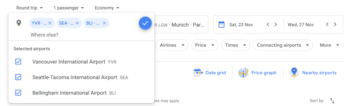This detailed caption describes a cluttered and text-heavy screenshot of a travel booking website:

The screenshot features a clean, white background at the top with menus for "Roundtrip," "One Passenger," and "Economy Class," each accompanied by corresponding drop-down options. A pop-up banner prominently appears on the left side of the image. 

Within the pop-up, there is a section organized by location; each location is denoted with a blue circle, containing a drop-down menu as well. The header of this section reads "Selected Airports" in bold, black text. A blue circle with a white check mark sits adjacent to this text. Below, an enumerated list of airports includes "Vancouver International Airport," "Seattle-Tacoma International Airport," and "Bellingham International Airport."

On the right side of the screenshot, the pop-up partially obscures some elements of the website. However, visible details include a calendar displaying specific dates: "Saturday, 23 November" and "Wednesday, 27 November." Additionally, there are drop-down menus labeled "Airlines," "Price," "Times," "Connecting Airports," and more.

Further down, the image reveals various graphics and text options such as "Nearby Airports," "Price Graph," and "Grid." Unfortunately, some of these elements are blurred and difficult to read clearly.